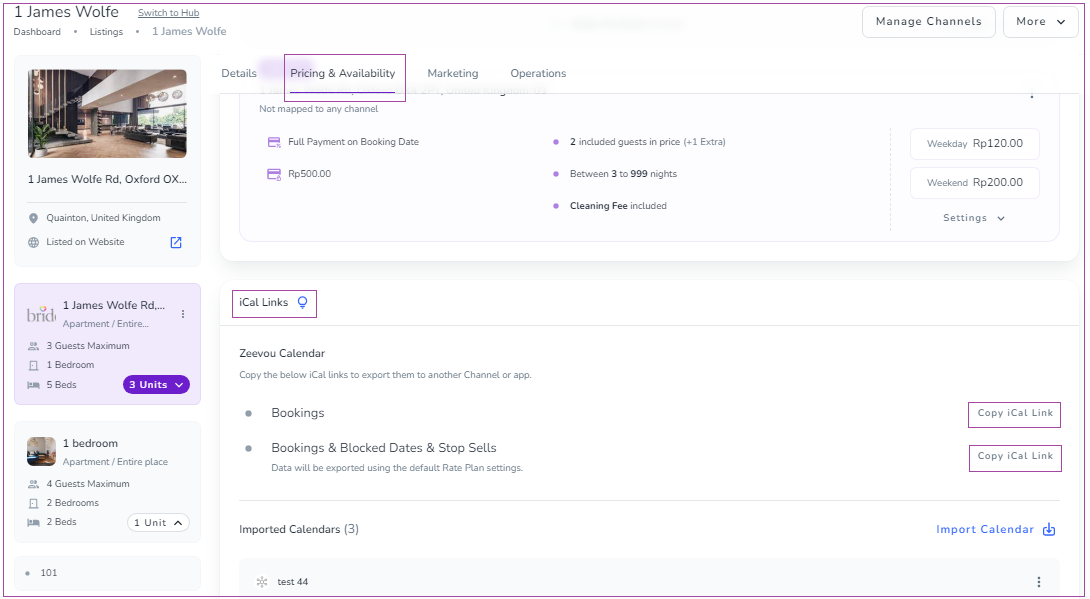This detailed image captures a webpage listing for James Wolfe, spelled W-O-L-F-E, located in Quantan, United Kingdom. The top section prominently displays his name along with navigation options such as "Dashboard," "Listings," and "Switch to Hub," the latter underlined for emphasis. The webpage has a predominantly white background with accents in purple and blue, notably for bullet points and clickable links.

A detailed section mentions that the apartment accommodates a maximum of three guests with one bedroom and five beds. Nearby, another listing states a different accommodation capacity: four guests with two bedrooms and two beds in one unit. Additional details include "Pricing and Availability," displayed with a purple line beneath it, and the notice "not mapped to any channel" accompanied by ICAL links.

The medium section reveals a clear image of the apartment, reinforcing the one-bedroom specification. Overall, the interface is clean and navigable, executed in a minimalist color scheme with strategic use of purple to highlight important links and sections.